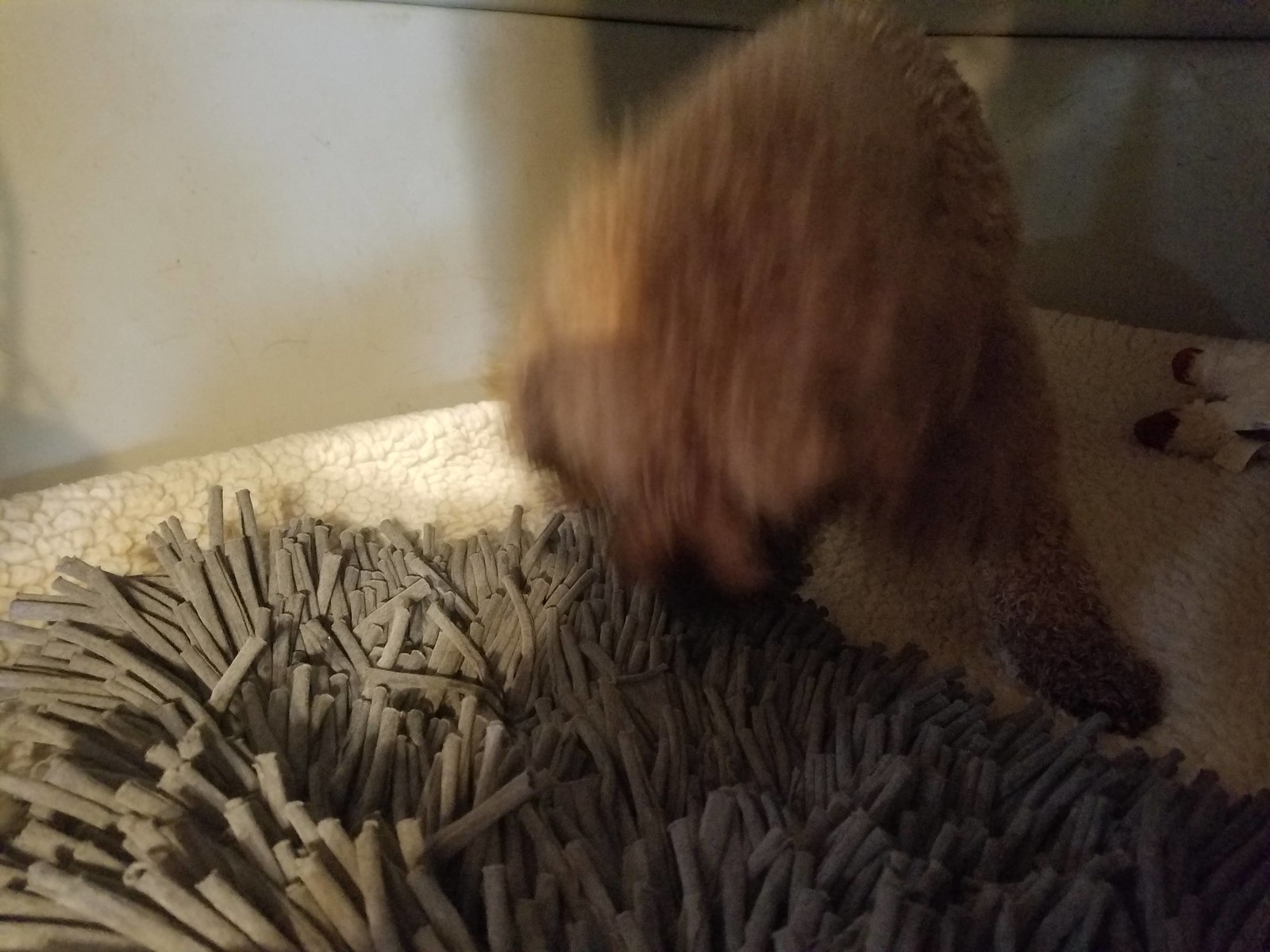A playful canine is captured with its face buried into a luxurious white fur carpet, creating an adorable scene of immersion. The background is minimalist, featuring white walls that enhance the overall brightness of the setting, which balances with the gentle shadows cast on the right side. Near the bottom left corner, patches of small, black, anemone-like fur add an intriguing and contrasting texture to the composition. The dog's white legs are partially visible, adding to the sense of depth and interaction within the environment.